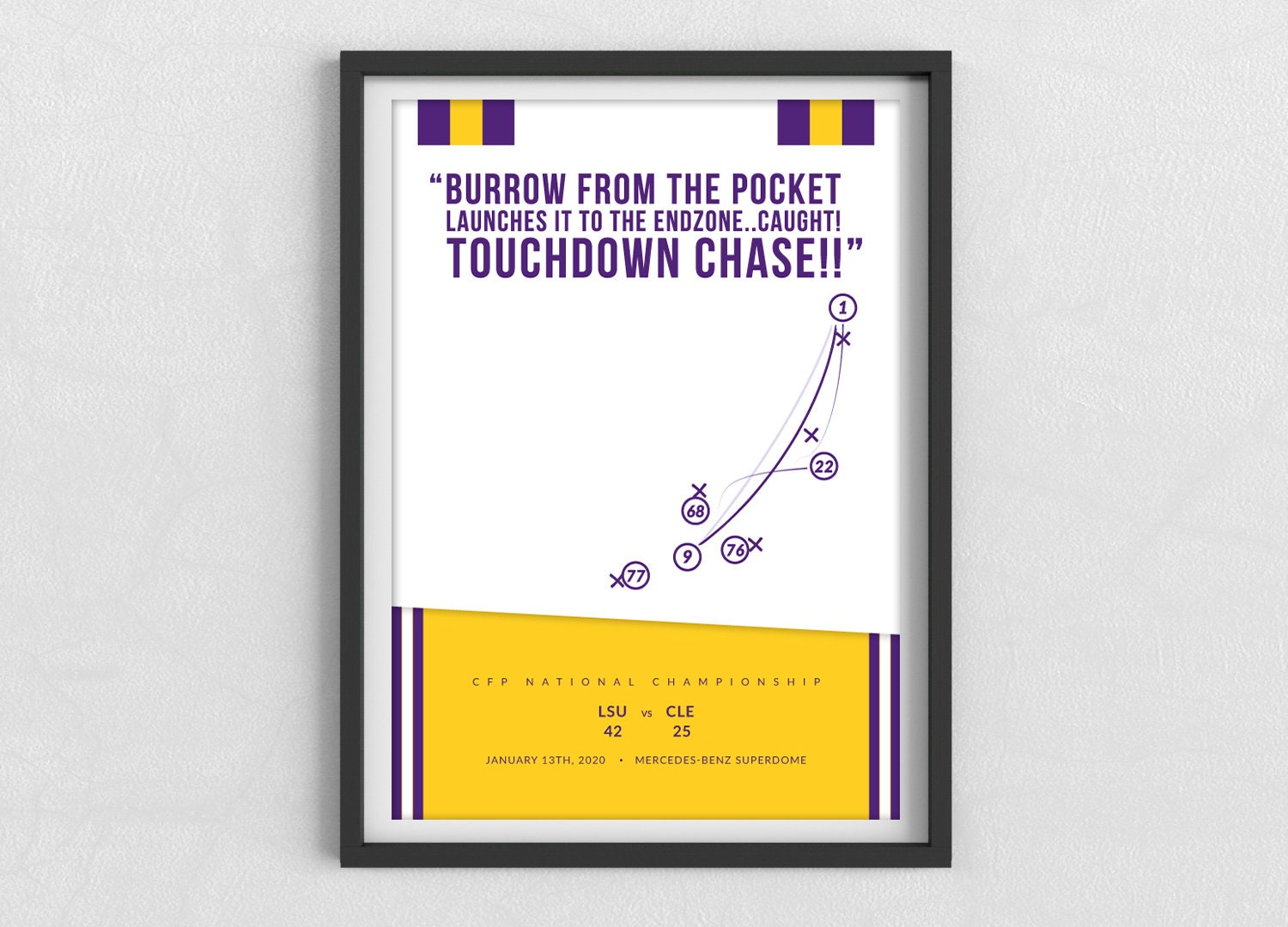The photograph captures a framed poster specifically designed for commercial use, set against a solid gray background to emphasize the product, commonly for online retail or catalog displays. The image is rectangular, oriented with the longer sides on the top and bottom. The main focus is a rectangular poster within a black wooden frame, featuring a gray inner border. The poster itself has a white background with notable purple and yellow accents indicative of LSU's team colors.

At the top, vertical stripes in black, purple, yellow, and purple adorn both the left and right corners, creating a header-like effect. Below this header, in purple all-capital text, the quote reads: "BURROW FROM THE POCKET. LAUNCHES IT TO THE END ZONE... CAUGHT! TOUCHDOWN, CHASE." The quote occupies the top two-thirds of the poster and is accompanied by a football diagram detailing player placements with circles, numbers, and directional lines.

The bottom third of the poster features a yellow placard with a purple border. In purple text, it states: "CFP National Championship, LSU vs. Clemson, 42-25, January 13th, 2020, Mercedes-Benz Superdome." This section commemorates LSU's victory in the championship game and adds context to the football diagram above. The clear, descriptive framing and elements make this poster a striking tribute to a memorable sports event.